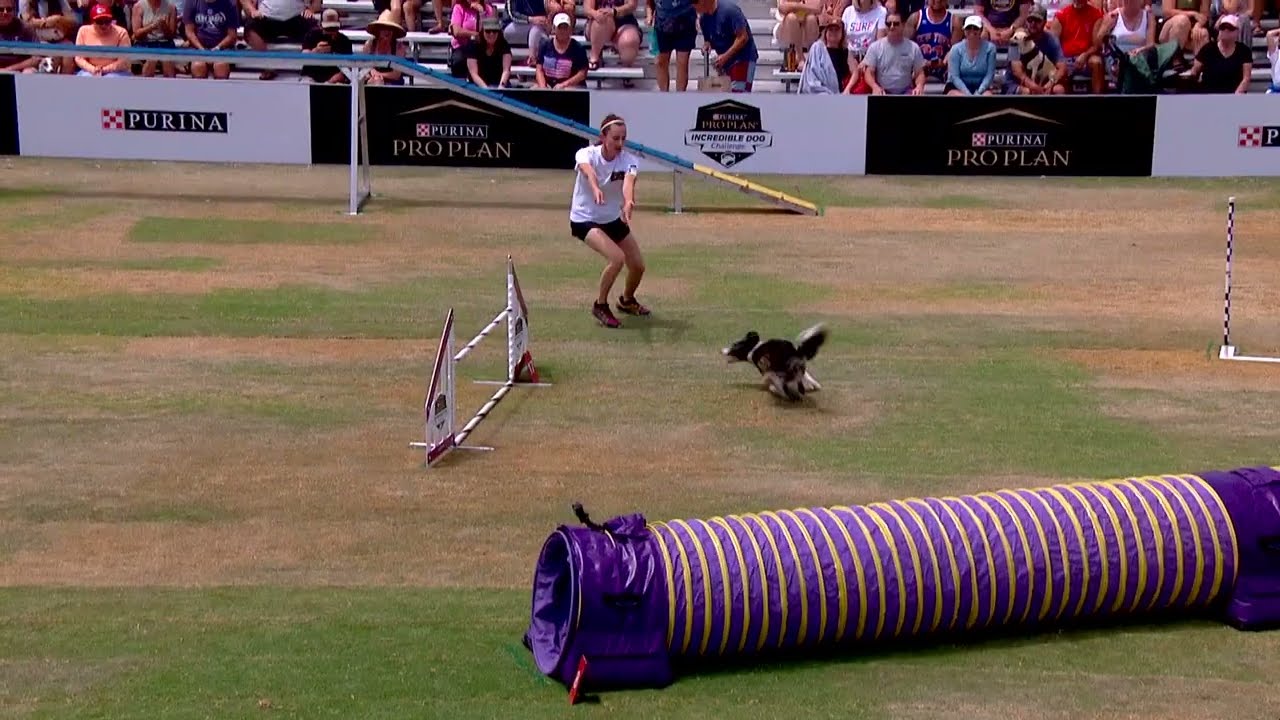This vibrant horizontal photograph captures an exciting moment during a dog agility contest. In the center of the image, a small black and white border collie is in mid-run, racing towards a jumping obstacle with focused determination. The dog's trainer, a young woman dressed in black shorts, a white shirt, a white headband, and black and red sneakers, is positioned to the top left of the dog. She uses animated hand gestures to guide it. The ground beneath the dog is a mix of patchy green and brown grass, suggesting a well-trodden field. A purple tube, presumably part of the obstacle course, is seen in the foreground, hinting at the dog's next challenge. The vibrant palette of purple and yellow obstacle equipment contrasts with the natural green grass. Billboards in the background prominently display sponsorship logos such as Purina and Purina ProPlan. The backdrop includes a bustling crowd of spectators in the bleachers, clad in black, blue, and gray shirts, many wearing hats, all intently watching the event. The scene is lively and detailed, encapsulating the excitement and coordination of a dog agility contest.